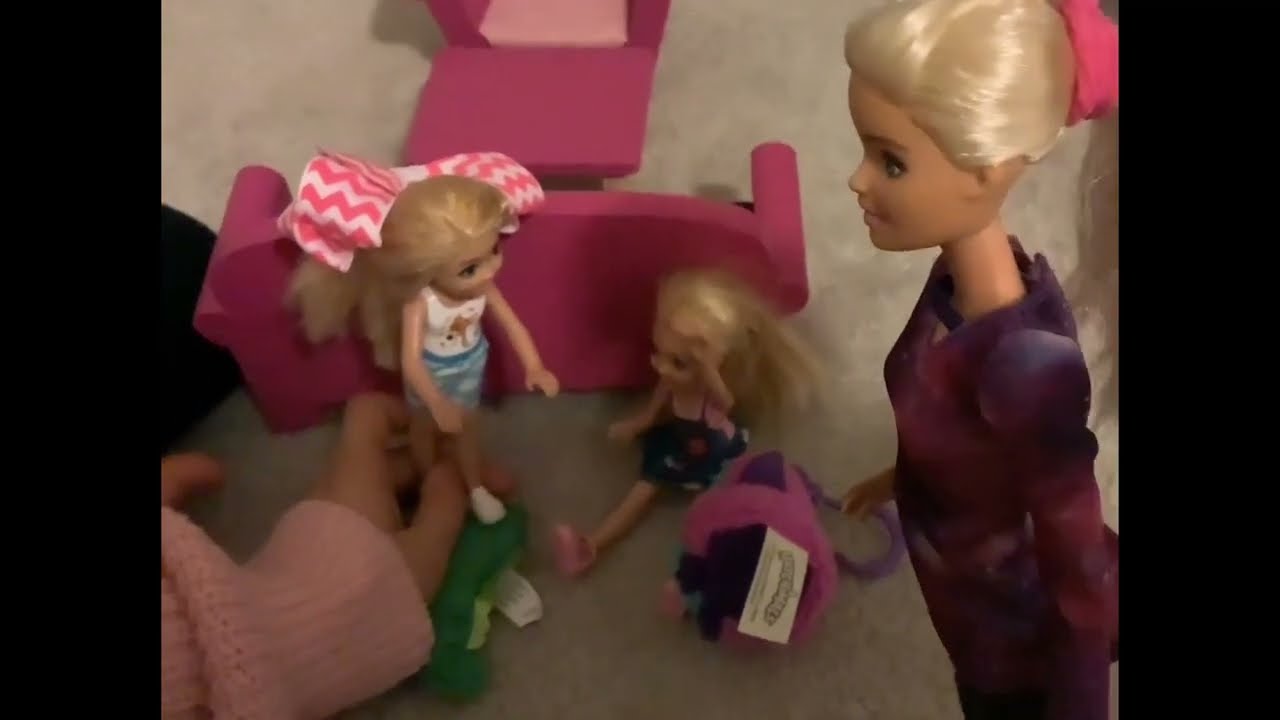In the center of the image, a group of Barbie dolls is set up in what looks like a child's play area. The scene features a blonde, adult Barbie doll on the right, dressed in a purple galaxy-patterned dress. This adult doll is accompanied by two smaller Barbie dolls, possibly representing children, dressed in shorts and playing beside a pink sofa. The setup is on a beige carpet, hinting at an indoor setting, likely a child's room.

To the left of the image, a human hand, likely a little girl's, reaches in from the bottom left corner, grasping one of the smaller dolls. The hand is clad in a pink long-sleeved sweater, adding a splash of color to the scene. In front of the pink sofa sits a small, pink side table, complemented by various colors throughout the scene, such as shades of blue, green, and white.

The arrangement, colors, and presence of the girl's hand provide a first-person perspective, making it seem like a candid moment captured during a child's imaginative playtime with her Barbie dolls.